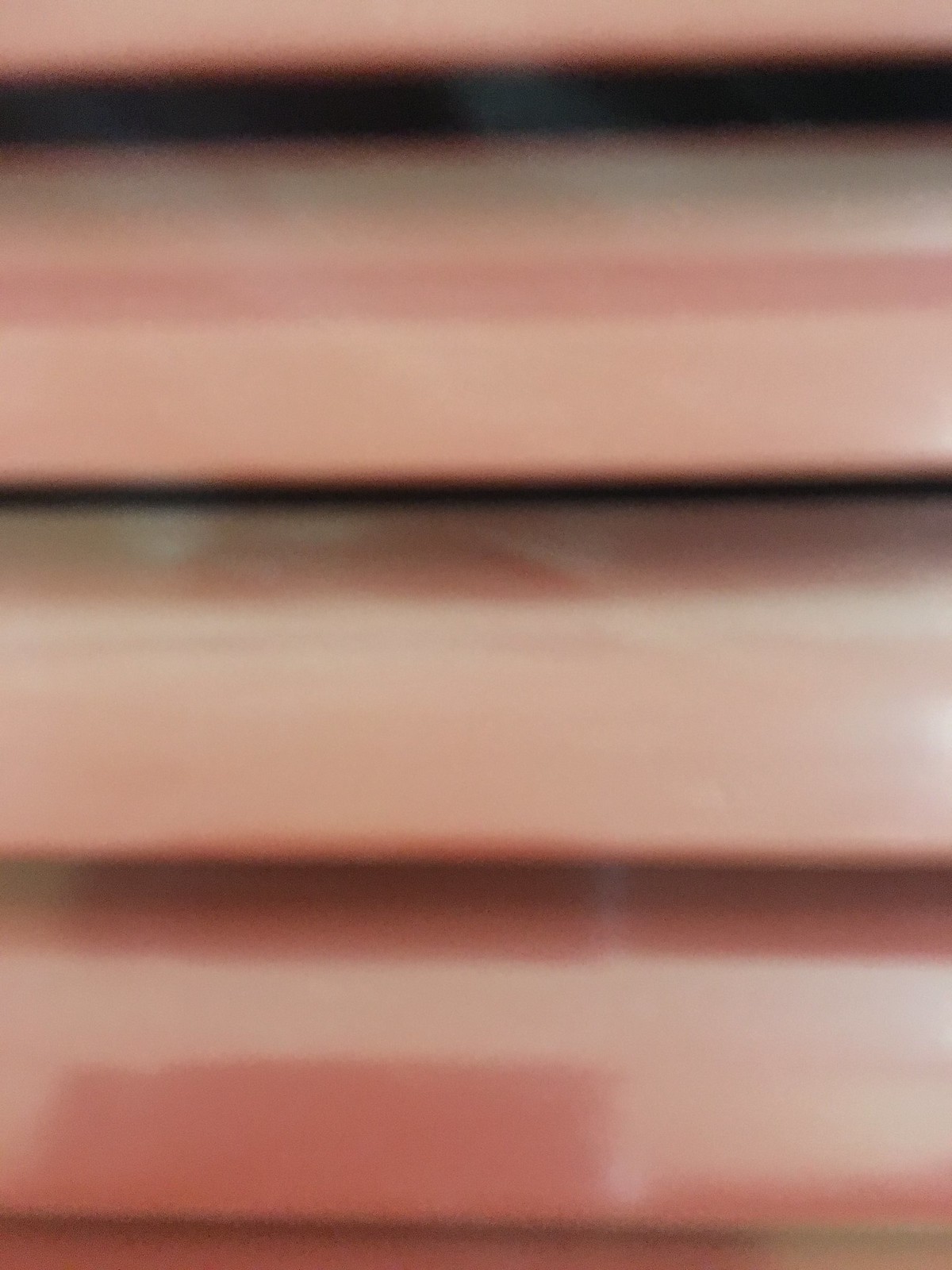This image is a very blurry, extreme close-up in a vertical, portrait mode format, capturing what seems to be overlapping horizontal slats or siding. Dominated by faded and sun-damaged shades of red and coral, the blurry photo lacks clear details but reveals some dust, stains, and shadow marks on the underside of the ridges. The image is brightened by sunlight, with reflective and lighter areas suggesting possible sun damage or faded paint. The slats, possibly cedar wood, appear to be at an approximate 65 to 70-degree angle, with noticeable gaps between them, making it difficult to discern the background. The whole screen is filled with these horizontal lines in varying shades of light pinkish-brown and darker reds, creating an indistinct yet textured visual.